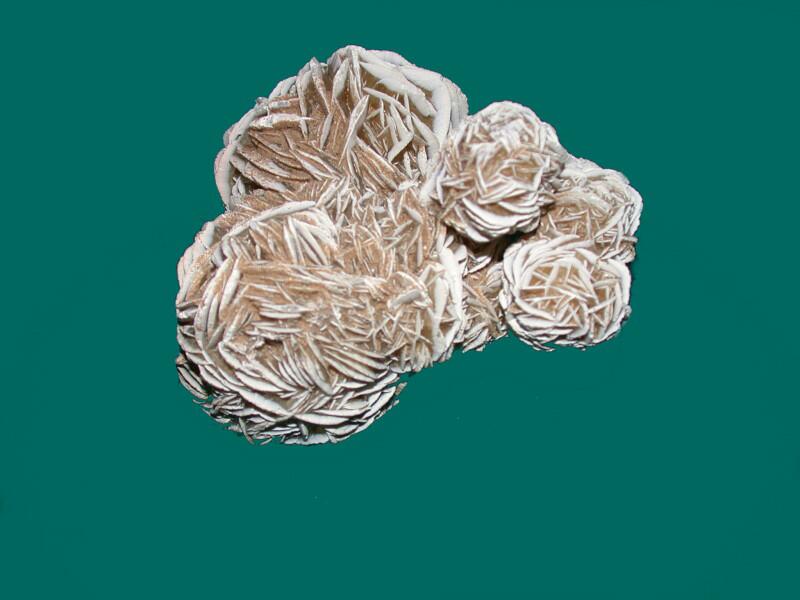This image displays an enigmatic object centered against a solid teal background, leaning slightly more towards green than blue. The main object, which occupies most of the image, is an intricate, textured structure with a mix of white and light brown hues. It resembles a crystalline or geode-like formation with a composition that suggests it might be stone, clay, or even fused seeds. The object features distinct circular clusters: three on the right side, a larger one on the left, and an even larger one at the bottom left, all seamlessly joined together. These clustered shapes evoke comparisons to a group of seeds, potentially a fruit or some type of natural formation. The entire image has a complex, almost organic feel, with the clustered circles providing a focal point amidst the structure’s rough, crystalline texture.